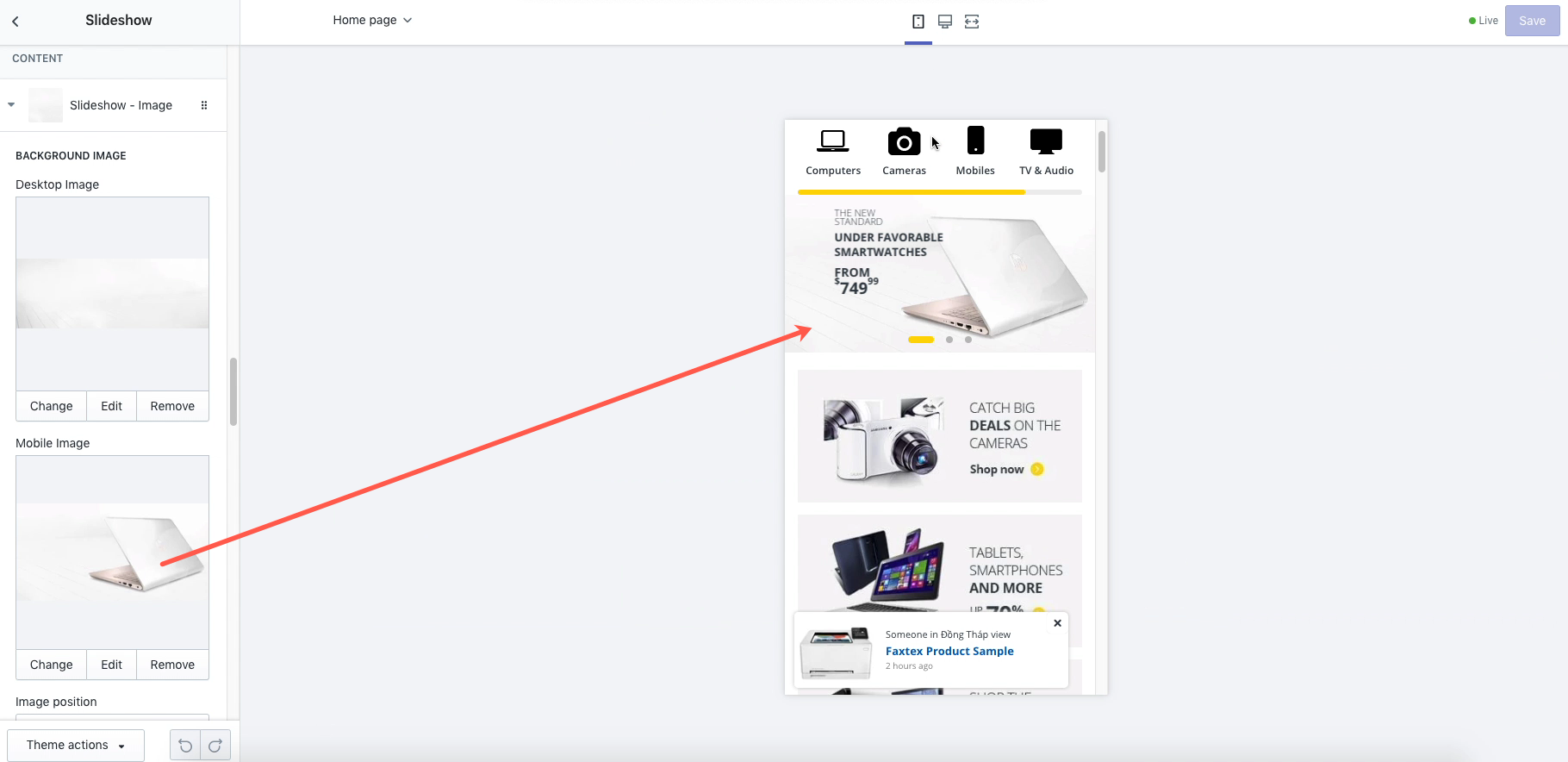This is a detailed screenshot of a slideshow program interface. In the top left corner, the word "Slideshow" is displayed in black font, accompanied by an arrow button to navigate back to the main page. Below "Slideshow," there's a vertical panel of options. At the top of this panel, it says "Content" in small gray font, followed by a dropdown box set to "Slideshow Image." Beneath the dropdown, "Background Image" is marked in bold small black font, and below that, "Desktop Image" is labeled in black font. A blank square thumbnail is displayed under "Desktop Image," with options to "Change," "Edit," or "Remove." Further down, "Mobile Image" is indicated next to a thumbnail displaying a side view of a laptop's backside. This thumbnail also has "Change," "Edit," or "Remove" options beneath it.

To the right of this vertical panel, the central section features a large gray background. Within this gray background, there's a mobile screenshot depicting an electronics store homepage. This homepage includes an advertisement with the same image of the laptop that is shown in the left panel. A red arrow icon points from the laptop image on the left panel to the corresponding image on the electronics store homepage, suggesting that this image can be saved and separately included in a slideshow.